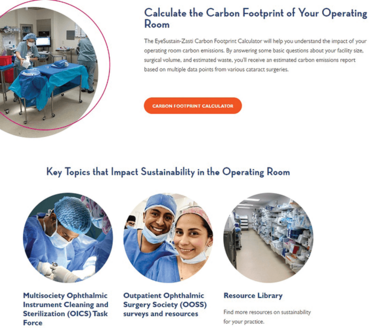This cropped screenshot features a detailed sustainability infographic tailored for hospitals, set against a clean white background. In the top left corner, there's a circular image of medical staff dressed in scrubs, working in an operating room. Adjacent to this image, to the right, small blue text reads, "Calculate the Carbon Footprint of your Operating Room." Beneath this line, even smaller blue text provides a brief description.

Below the description, there’s an orange button labeled "Carbon Footprint Calculator" in white print. Further down and centered near the bottom of the screenshot, bold text states, "Key Topics that Impact Sustainability in the Operating Room." Directly underneath, three circular thumbnail images are displayed horizontally:

1. The first thumbnail shows a surgeon actively performing an operation.
2. The second depicts two doctors in scrubs taking a selfie.
3. The third features a neatly organized stock room for operating supplies.

Accompanying these images are concise descriptions. Beneath the surgeon image, the text lists: "Multi-Society Ophthalmologic Instrument Cleaning and Sterilization Task Force, Outpatient Ophthalmologic Surgery Society, Surveys and Resources," and then, "Resource Library."